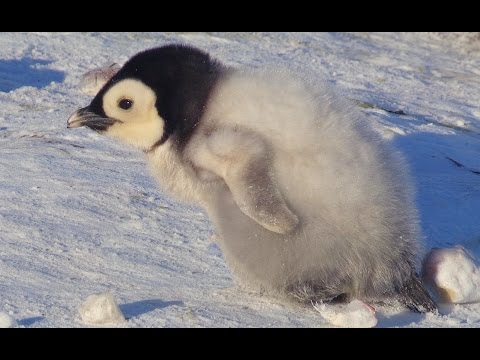This is an image of an adorable, fluffy baby penguin standing on a snow surface under a low-quality, warm light, suggesting it's near sunrise or sunset. The small penguin, slightly hunched over and looking to the left of the frame, is covered in downy, gray fur on its tummy and back, with contrasting black and white features on its head. It has a distinctive black head with white patches around its black eyes, and a beak that transitions from dark gray at the base to white at the tip. The scene includes slight shadows and a few snowballs scattered around the penguin, with a black border framing the image top and bottom. The overall snowy background possesses a yellowish and bluish hue due to the lighting, enhancing the serene yet captivating moment captured.